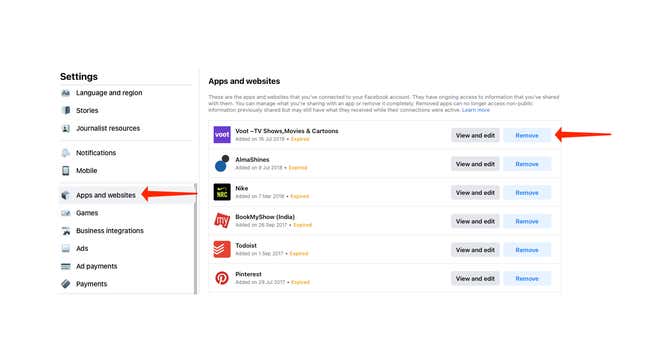The image is a screenshot of a settings page divided into two sections. On the left-hand side, at the top, the title "Settings" is displayed in black. Below this, a thin gray horizontal line separates the title from the menu options listed underneath: "Language & Region," "Stories," "Journalists," and "Resources." Another thin gray line appears further down, with the options "Notification," "Mobile," "Apps," and "Websites" highlighted in gray. A red arrow points to this section, indicating its importance. Other options listed include "Games," "Business Integrations," "Ads," "Ad Payments," and "Payments."

A vertical gray line separates this left section from the right section. At the top of the right section, the title "Apps and Websites" is written in black, although it appears somewhat blurred and difficult to read. Below this title, additional text is mostly unreadable except for a blue hyperlink that says "Learn More."

Further down in the right section, a list of items is visible: "Root, TV Shows, Movies, and Cartoons," followed by "Nuke," "Book My Show," "Do This," and "Pinterest." Each of these items is accompanied by two rectangular buttons. The first rectangle is gray, with "View and Edit" written in black, and the second rectangle is light blue, with "Remove" written in darker blue. A red arrow points specifically to the "Remove" button next to "Root, TV Shows, Movies, and Cartoons," emphasizing this option for an unknown reason.